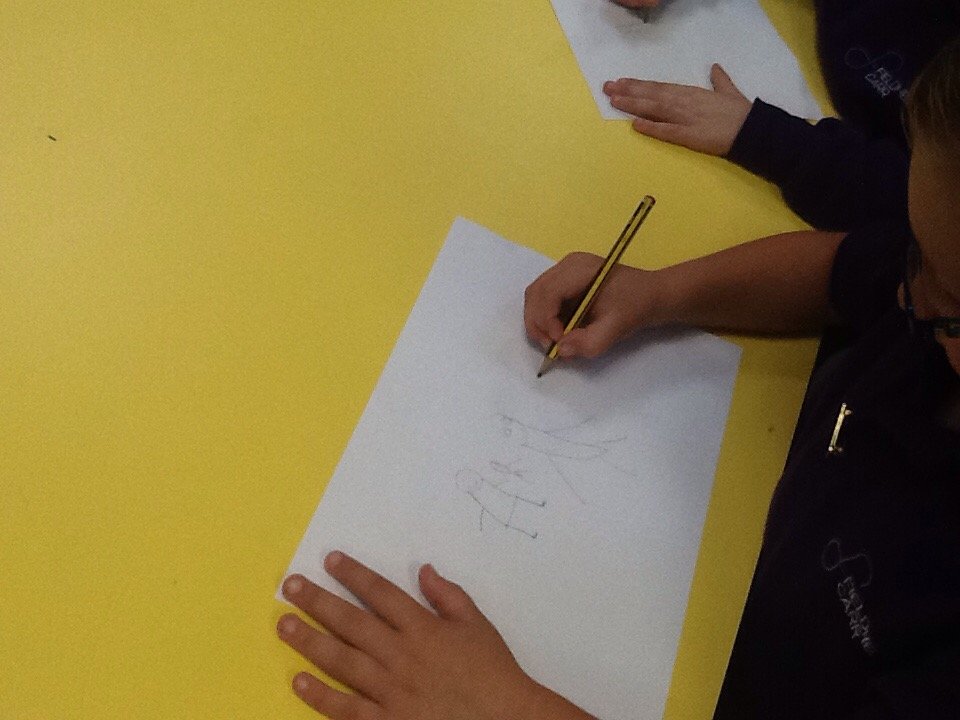This color photograph features a top-down view of two people drawing on a bright yellow table. The central focus is a man, likely with a Latino or Middle Eastern skin tone, wearing a navy blue shirt. His left and right hands are engaged as he draws stick figures on a white rectangular piece of paper. The man holds a gold-plated pencil in his right hand. His drawing includes three stick figures, arranged in a manner suggestive of a family: a medium-sized figure on the left, a smaller figure in the center, and a larger figure on the right. 

In the upper right corner of the image, we see the left hand of another person with a slightly lighter skin tone, possibly a child. This person, dressed in dark-colored attire—navy blue or black—holds down another piece of white paper. The partial view of their forehead and knuckles hints that they, too, are focused on their own drawing activity. The apparent simplicity of the stick figures, combined with the collaborative scene, evokes a sense of casual creativity, reminiscent of a child's doodling session.